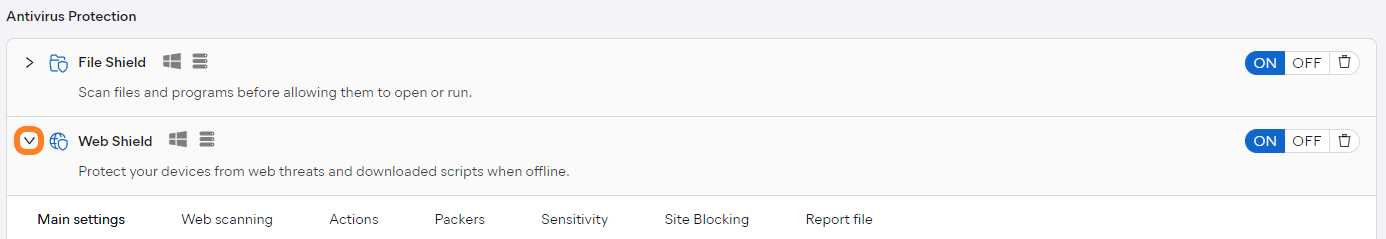The image captures the top section of a web page screenshot focusing on antivirus protection settings. The bottom portion of the web page is blank and entirely white, without a border. The header bar at the top is a very light gray color, and it has the text "Antivirus Protection" displayed on the upper left-hand corner.

Below the header bar are two horizontal boxes. The first horizontal box begins with a right arrow followed by a blue icon labeled "File Shield." Accompanying this icon are two smaller icons. The description under "File Shield" reads, "Scan files and programs before allowing them to open or run."

The second horizontal box, located underneath, features an orange circled down scroll button accompanied by a blue icon labeled "Web Shield." Next to and under this icon are two gray icons. The description under "Web Shield" states, "Protect your device from web threats and downloaded scripts when offline."

Both horizontal sections include an "On/Off/Delete" switch on the right-hand side. In this screenshot, the "On" option is highlighted in blue within both sections.

At the bottom of the captured section is a toolbar with seven tabs listed from left to right: Main Settings, Web Scanning, Actions, Packers, Sensitivity, Site Blocking, and Report File. The "Main Settings" tab is highlighted in darker black text, indicating it is the currently selected tab.